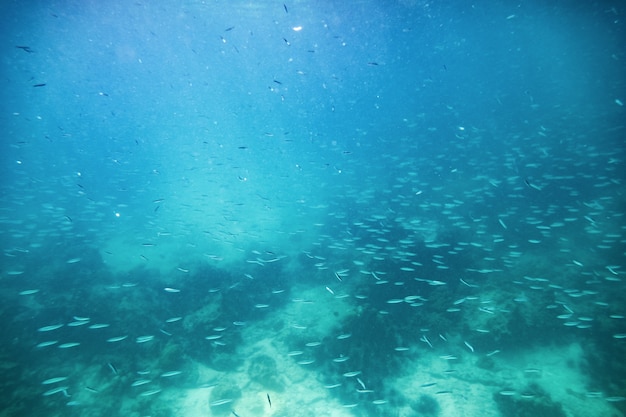This underwater image captures a vibrant, slightly blurry scene bathed in a turquoise blue hue. Illuminated by sunlight filtering down from the top left corner, the light casts a glow that highlights the small, white, darting fish, likely minnows, that populate the scene. These fish, some moving together in one direction while a few swim perpendicularly, contrast against the ocean floor adorned with sporadic clusters of seaweed or green plants. The sandy bottom, interspersed with rocks, appears partially stirred up, creating a cloudy, unfocused patch. Despite the overall slight fuzziness due to the water, the image effectively conveys the dynamic, bustling underwater environment.